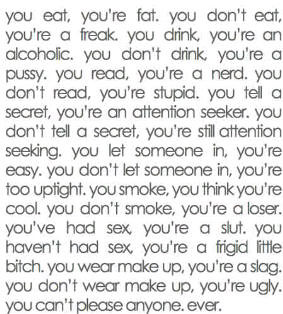The image predominantly features a series of lowercase text in light blue on a white background, closely arranged and spanning the entire frame. The text is a collection of judgmental statements formatted consistently with commas separating actions from insults and periods ending each sentence. The statements include: "you eat, you're fat. you don't eat, you're a freak. you drink, you're an alcoholic. you don't drink, you're a pussy. you read, you're a nerd. you don't read, you're stupid. you tell a secret, you're an attention seeker. you don't tell a secret, you're still an attention seeker. you let someone in, you're easy. you don't let someone in, you're too uptight. you smoke, you think you're cool. you don't smoke, you're a loser. you've had sex, you're a slut. you haven't had sex, you're a frigid little bitch. you wear makeup, you're a slag. you don't wear makeup, you're ugly. you can't please anyone, ever." The image encapsulates the relentless and contradictory nature of societal judgments aimed at individuals, leaving a powerful message about the impossibility of satisfying everyone.